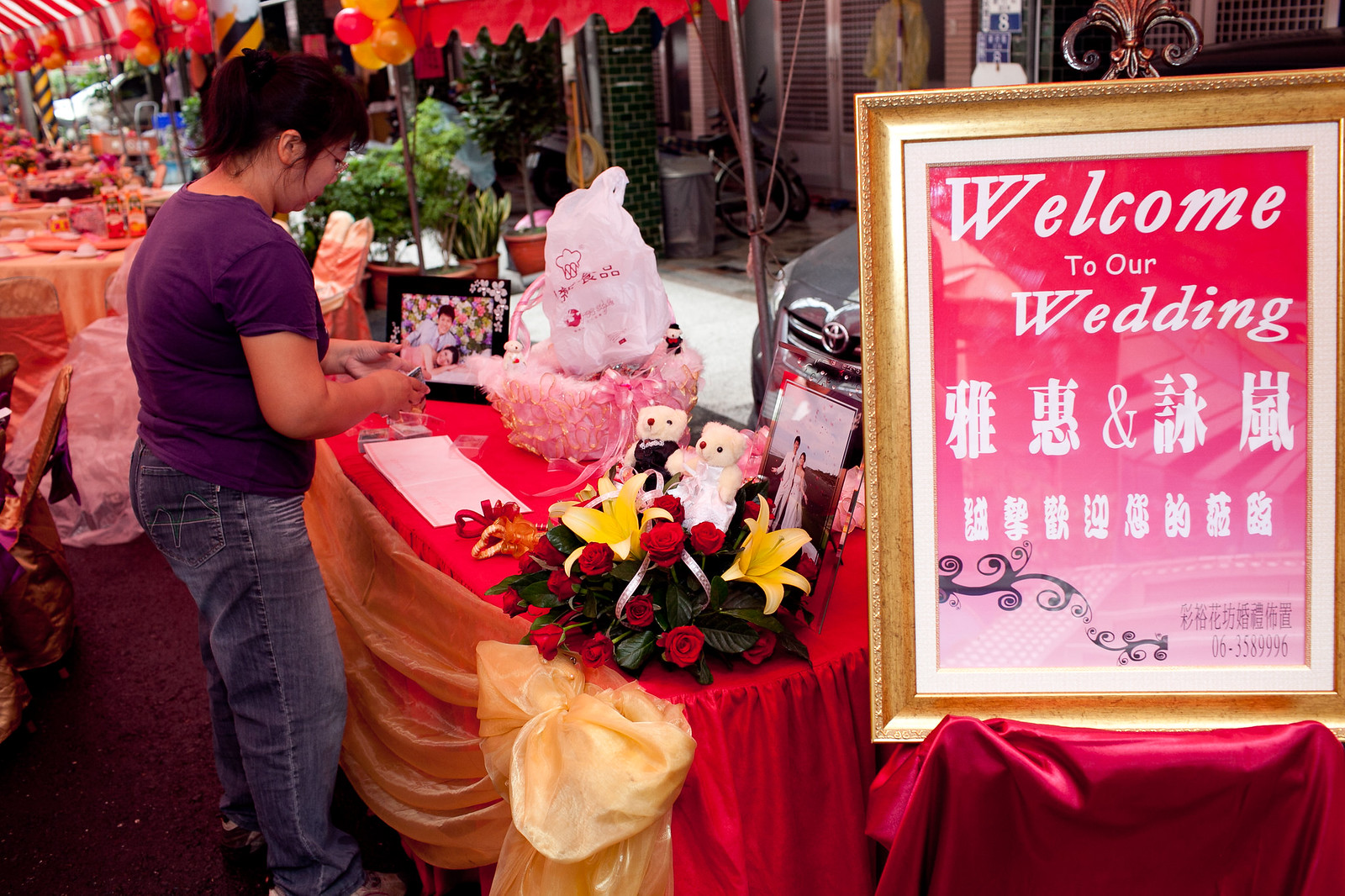The photograph captures a formal event set in an open-sided pavilion or tent, with visible surroundings including a parked car, houses, and businesses in the background. The left side of the image shows several round tables draped in orange tablecloths and set with tableware such as plates and napkins. In the center, there's a rectangular table adorned with a red tablecloth overlaid with a silk yellow cloth at the front. This table features a picture of a couple on both ends and a vibrant red rose floral arrangement topped with two teddy bears in the middle. To the right of the table stands a large framed sign with a pink background, white Asian characters, and the welcoming message "Welcome to Our Wedding."

A woman with medium-length black hair, wearing a short-sleeved blue or purple shirt and blue jeans, stands in front of this table, looking down. Her hands are positioned out in front of her. In the distance to the left, additional tables or counters are visible, laden with various items, while to the right of these tables, a sidewalk or street can be seen, adding depth to the setting. The overall atmosphere suggests a festive celebration, likely a wedding, with meticulously arranged decorations and intimate details.